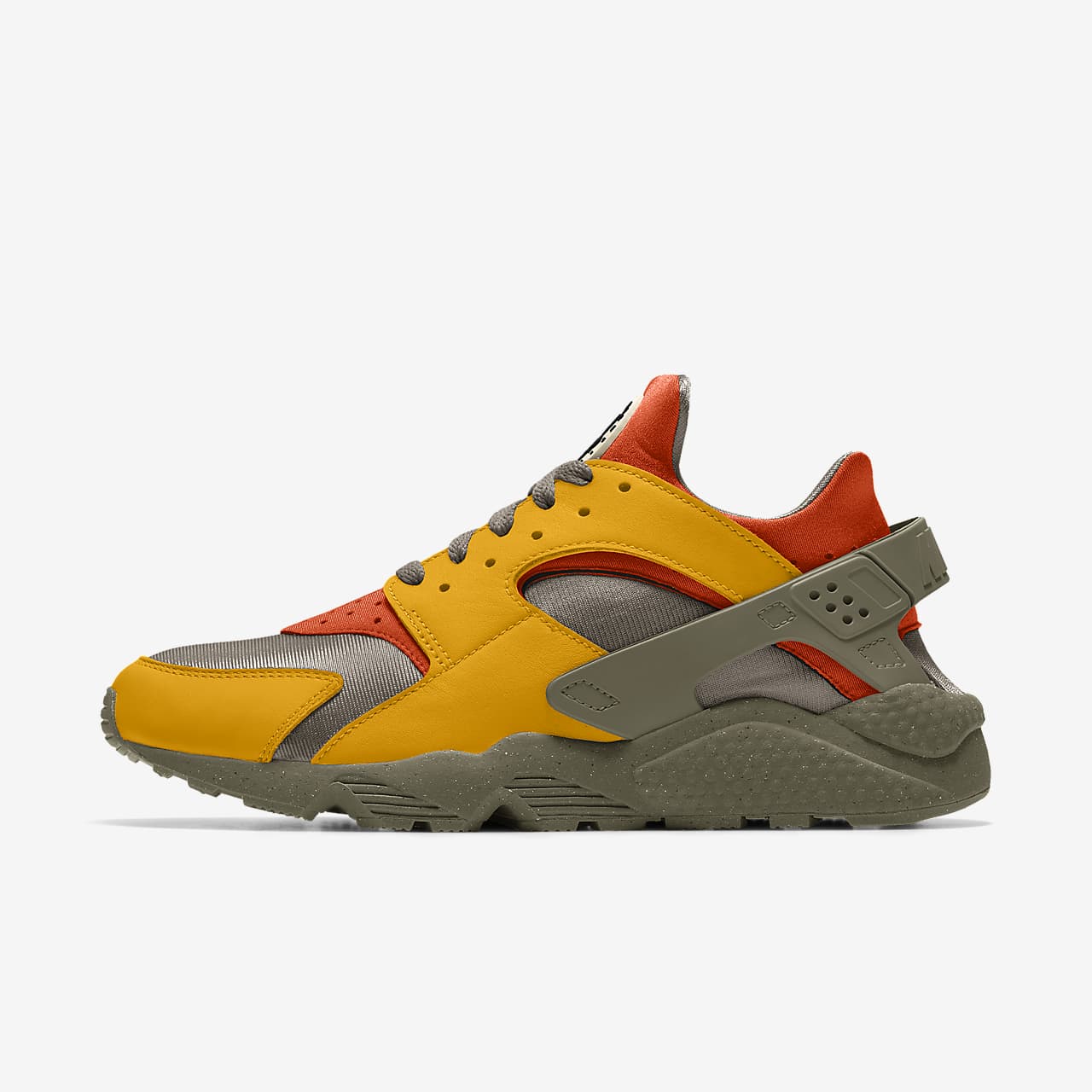This is a detailed profile photograph of an athletic sneaker, positioned with its heel on the right and toe facing left. The sneaker rests on a white surface, contrasting sharply against a white background. Its design appears futuristic and versatile, suitable for both genders. The sneaker features a thick, grey, treading sole designed for running and gripping various surfaces, becoming thinner towards the toe and thicker at the heel for enhanced support. The shoe combines multiple materials: a grey fabric body that resembles canvas, complemented by grey shoelaces and an adjustable plastic-looking grey strap around the ankle. Accents of yellow and orange leather are prominently seen around the shoelaces and sides, with a distinctive red band near the ankle opening. Small yet attentive stitching in red and brown decorates the structure, enhancing its sturdy yet stylish appeal. The image, devoid of any text, would fit perfectly on retail websites like Foot Locker or Nike, showcasing the sneaker's modern and athletic design.